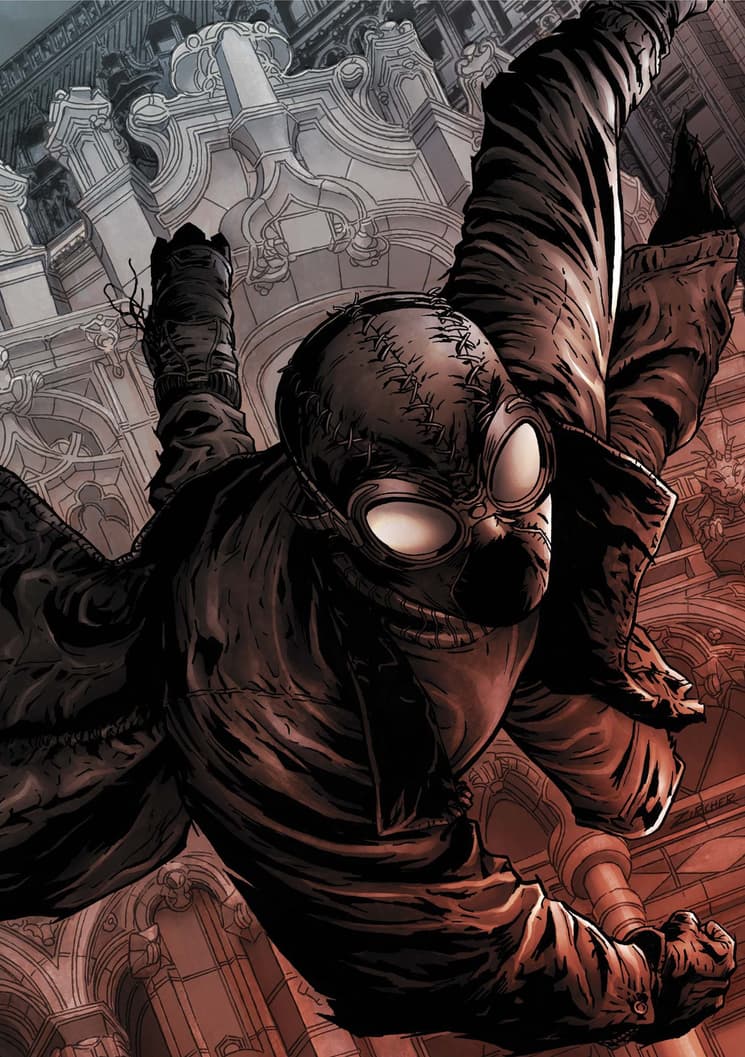This comic book-style illustration features a dark, enigmatic character reminiscent of Spider-Man, adorned with a distinctive goggled mask characterized by beetle-like eyes and multiple crisscrossed patchwork stitches—one above each eye and one above the nose. Dressed in a long, black, raggedy coat and gloves, the figure's dynamic pose takes center stage as they appear to be in motion, perhaps jumping, climbing, or gliding through the air. Architectural details, possibly resembling a church or cathedral, frame the backdrop, enhancing the sense of movement across the scene. The color palette transitions from gray in the upper left to shades of light gray, brown, black, and culminates in a red rust tint at the lower right, adding depth and energy to the image. Black, untied boots and threads hanging from the clothing further emphasize the character's gritty, action-packed appearance.